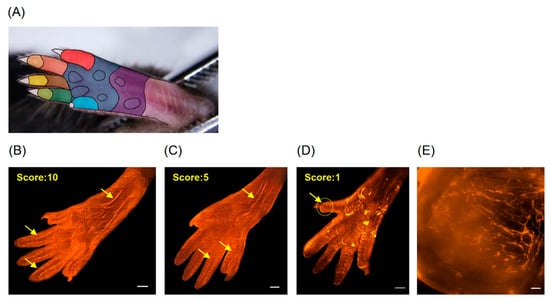This is an image series consisting of five pictures, labeled A through E. Picture A, located at the top left and rectangular in shape, features a vividly painted hand or possibly an animal paw. The hand is adorned with various colors: the thumb is red with a white, pointy nail; the index finger is orange with a shaded gradient; the middle finger is green; the ring finger is brown with yellow; and the pinky is blue. The forearm has three wavy, horizontal bands—purple, blue, and pink—painted across it. The hand is positioned between two metal rails or strips. Below and to the right of picture A are four smaller, square images labeled B through E. These images resemble X-rays or infrared photographs of the hand. 
- Picture B, showing a predominantly red hand with a black background, is labeled with a score of 10 and features arrows pointing to the forearm and two fingers.
- Picture C, with a score of 5, displays a similar red hand with arrows directed at the wrist, thumb, and index finger.
- Picture D, scored 1, focuses on the thumb, marked by a single arrow.
- Picture E, unlike the others, is an orange blob against a black background, devoid of identifiable hand features.

The vivid colors and detailing on the hand in picture A contrast with the monochromatic, clinical presentation of pictures B, C, D, and E, which use arrows to highlight specific areas on the hand or paw. The images create a juxtaposition between artistic representation and scientific analysis.